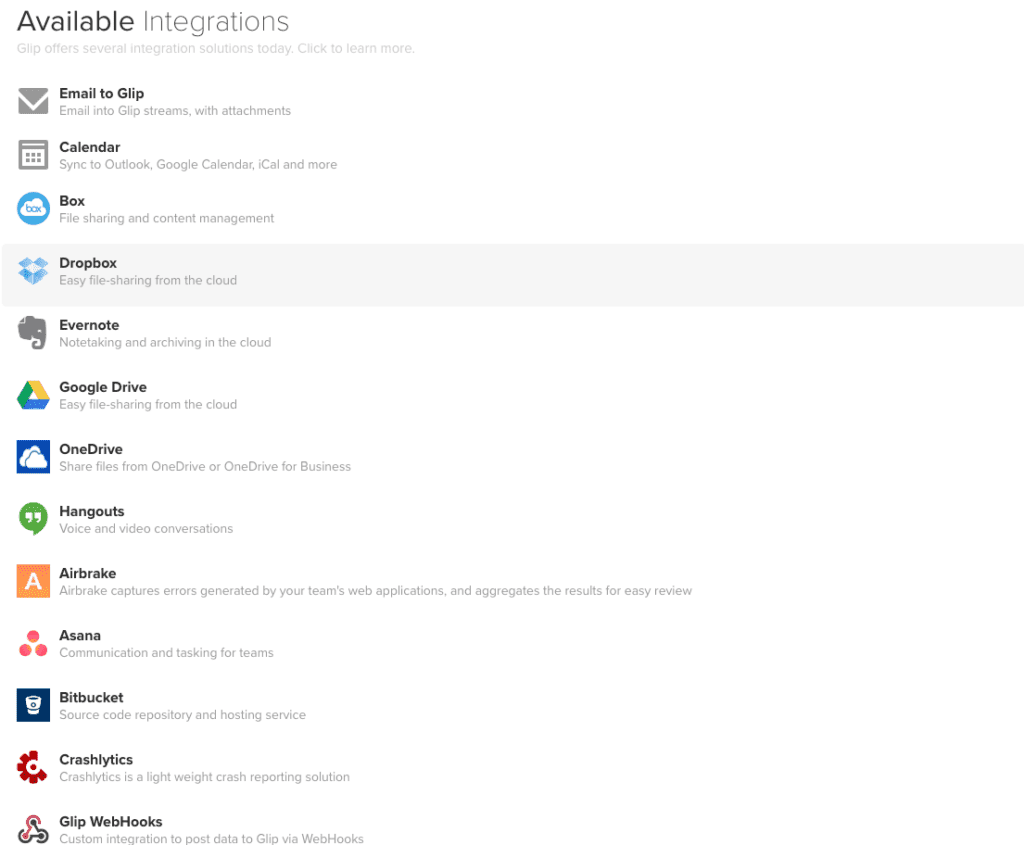The image displays a user interface section titled "Available Integrations," where "Available" is prominently highlighted in bold black text, and "Integrations" is in a lighter gray color. Beneath this header, a smaller font reads: "GRIP offers several integration solutions today. Click to learn more."

Below this text, various integration categories are listed:

1. **Email to GRIP and Email to GRIP Streams with Attachments**: Accompanied by a small gray envelope icon, indicating email integration options.
2. **Calendar Sync**: This section includes options like Outlook, Google Calendar, iCal, and more, denoted by a calendar icon to the left.
3. **Box**: Labeled as "file sharing and content management," this category includes an appropriate icon.
4. **Other Integrations**: 
    - Dropbox
    - Evernote
    - Google Drive: Marked by its distinctive green, yellow, and blue logo.
    - OneDrive
    - Hangouts
    - Airbrick
    - Asana
    - Bitbucket
    - Crashlytics
    - Glip
    - Webhooks

Each integration is paired with its respective icon on the left side, making the list visually informative and easy to navigate.